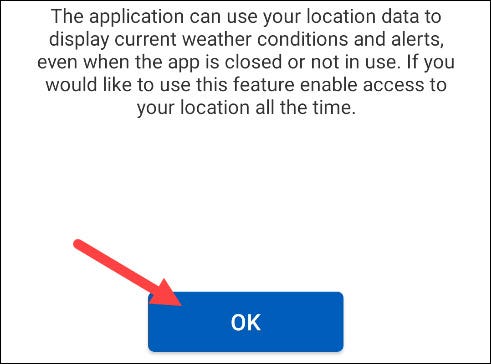The image showcases a notification box with a distinctive design and explicit instructions for the user. The notification box is bordered in black with a white interior, and prominently outlines the box's structure in black. The text within the box informs users about a feature of an application that utilizes location data to provide real-time weather information and alerts, even when the application is not actively in use. Users are prompted to enable this feature by allowing the app to access their location at all times. A large, rectangular blue button labeled "OK" is prominently featured within the notification, designed to capture the user's attention and encourage them to enable location access. An oversized red arrow directs the viewer towards this "OK" button, emphasizing the action required to activate the location-based weather updates and alerts.